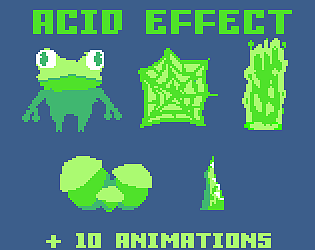The artwork is a square piece with a dark cornflower blue background, featuring lime green pixelated graphics reminiscent of early video game design. The top of the image displays the bold, video game-style text "ACID EFFECT" in bright green. Below, on the left, is a three-tone green frog standing upright with wide eyes and hands by its sides. In the center, there's a pixelated spider web. On the right is another green pixelated structure, which resembles flames. Towards the bottom left are shapes that look like pots filled with coins, although the green tones make this ambiguous. To the right of these pots is a pointed green rock shape. At the bottom of the image, the text "PLUS TEN ANIMATIONS" is displayed in the same bright green, video game-like font. The overall design is crudely made, with a color palette dominated by various shades of green and white.